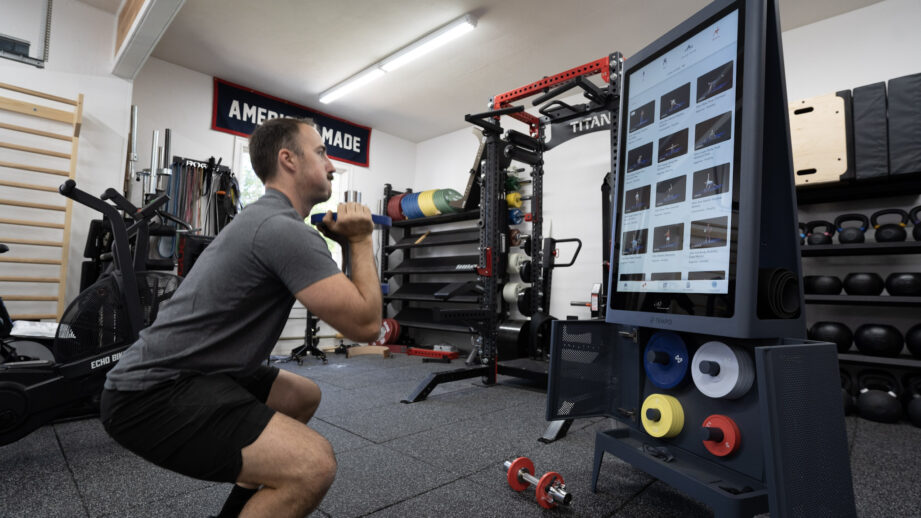The image captures a well-equipped gym, possibly professional, adorned with various workout equipment including racks of kettlebells, dumbbells, and weight plates in blue, silver, yellow, and red. Prominently, a middle-aged Caucasian man with a mustache is in the midst of performing a squat, while holding a blue weighted plate under his chin. He's dressed in a gray shirt and black shorts, positioned in front of a large workout mirror screen displaying a fitness class. Behind him, there are weight plates and kettlebells neatly arranged, with a striking red and black Titan squat machine visible. To his right stands an elliptical machine branded Echo. The gym's atmosphere is marked by white ceilings and walls, and a charcoal gray, interlocking floor with a bit of give. A black sign with red edges and white capital letters proclaiming “American Made” is affixed to one of the back corners of the gym. In front of the man, a dumbbell with red weights lies on the ground.